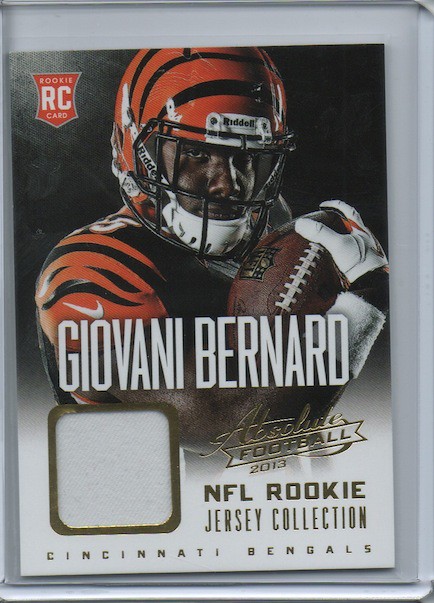The image is a football card featuring Giovanni Bernard from the Cincinnati Bengals, designated as a rookie card with an "RC" emblem over his left shoulder. The background is a white silver color, highlighting the memorabilia itself. Bernard is depicted prominently in his orange and black tiger-striped helmet and jersey, with a white chin guard and a white glove on his right hand, holding a football in his right arm. The text "Giovanni Bernard" is written in bold white letters across the middle of the card. Below, in gold font, it reads "Absolute Football 2013 NFL Rookie Jersey Collection" and "Cincinnati Bengals." A white square bordered in gold trim features a piece of Bernard's actual game-worn jersey. The card, protected by a card holder, is recognized as a relic card, making it a valuable piece of sports memorabilia for collectors.